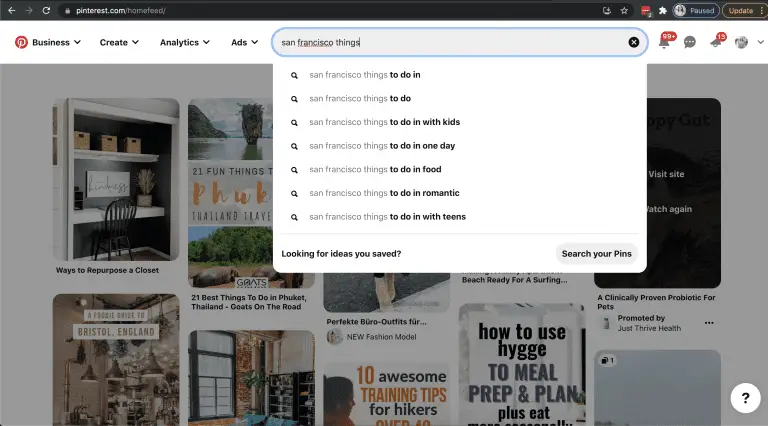The image is a screenshot of a Pinterest business account interface. In the upper left-hand corner, the distinctive red and white 'P' Pinterest logo is clearly visible. Adjacent to it, a row of drop-down menus labeled 'Business,' 'Create,' 'Analytics,' and 'Ads' can be seen. The search bar at the top contains the phrase "San Francisco things," and the predictive text offers several suggestions, such as "San Francisco things to do in," "San Francisco things to do," "San Francisco things to do in with kids," "San Francisco things to do in one day," "San Francisco things to do in food," "San Francisco things to do romantic," and "San Francisco things to do with teens."

Directly under the search bar, there is an option labeled "Looking for ideas you saved? Search your pins," indicating a drop-down menu for further navigation. Below this is the main content area, laid out in a grid of rectangular image cards typical of Pinterest. The first image on the left depicts a desk built into the wall with accompanying shelves and a chair positioned in front. Some visible labels beneath the images include "How to use hygiene to meal prep and plan plus eat," and "10 awesome training tips for hikers." Although many of the other labels are not clear, the familiar layout and design elements confirm this is indeed a Pinterest page.